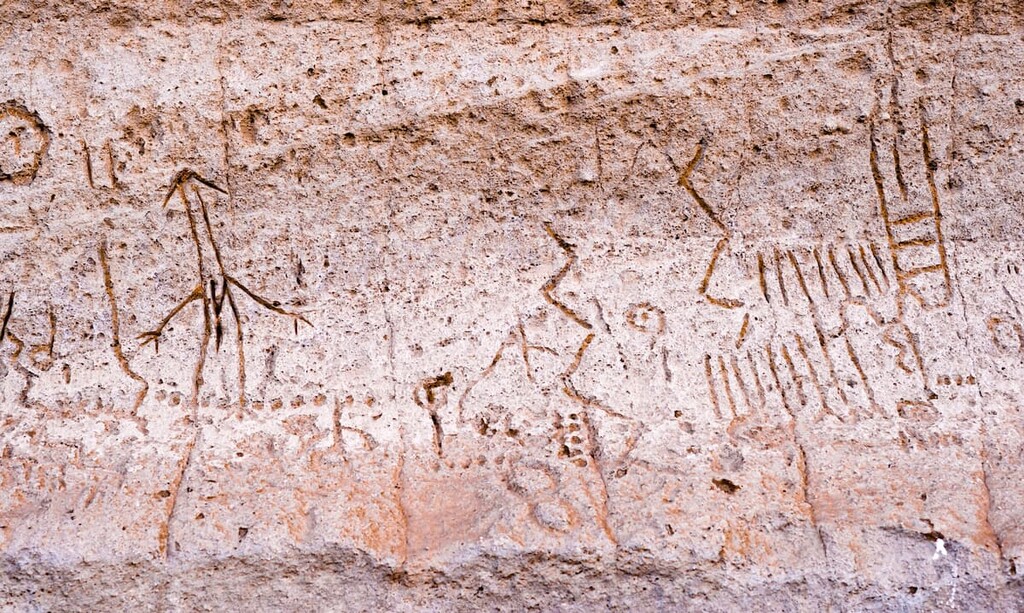The image captures the inner wall of what appears to be a cave or an ancient stone structure. The stone surface is a mosaic of various shades of browns, oranges, and creams, with regions exhibiting rust-like and orange hues, especially toward the bottom. The wall is covered in numerous distinct carvings and etched drawings. Prominent among these are various geometric shapes such as circles, zigzags, and arrows pointing in different directions. Numbers, including a notable number 8, several clusters of dots, and sequences of short lines, are also carved into the stone, suggestive of counting or tallying. There's a human stick figure with two arms and legs, and in the center, complex zigzag patterns dominate. The left side showcases circles and possibly faces simply depicted with two eyes and a line for a mouth. The carvings, characterized by their bold lines, could be remnants of an ancient script or pictographs, potentially telling a story or bearing symbolic meanings. The overall appearance suggests that these artworks are quite old, possibly indicating an ancient form of communication or record-keeping.